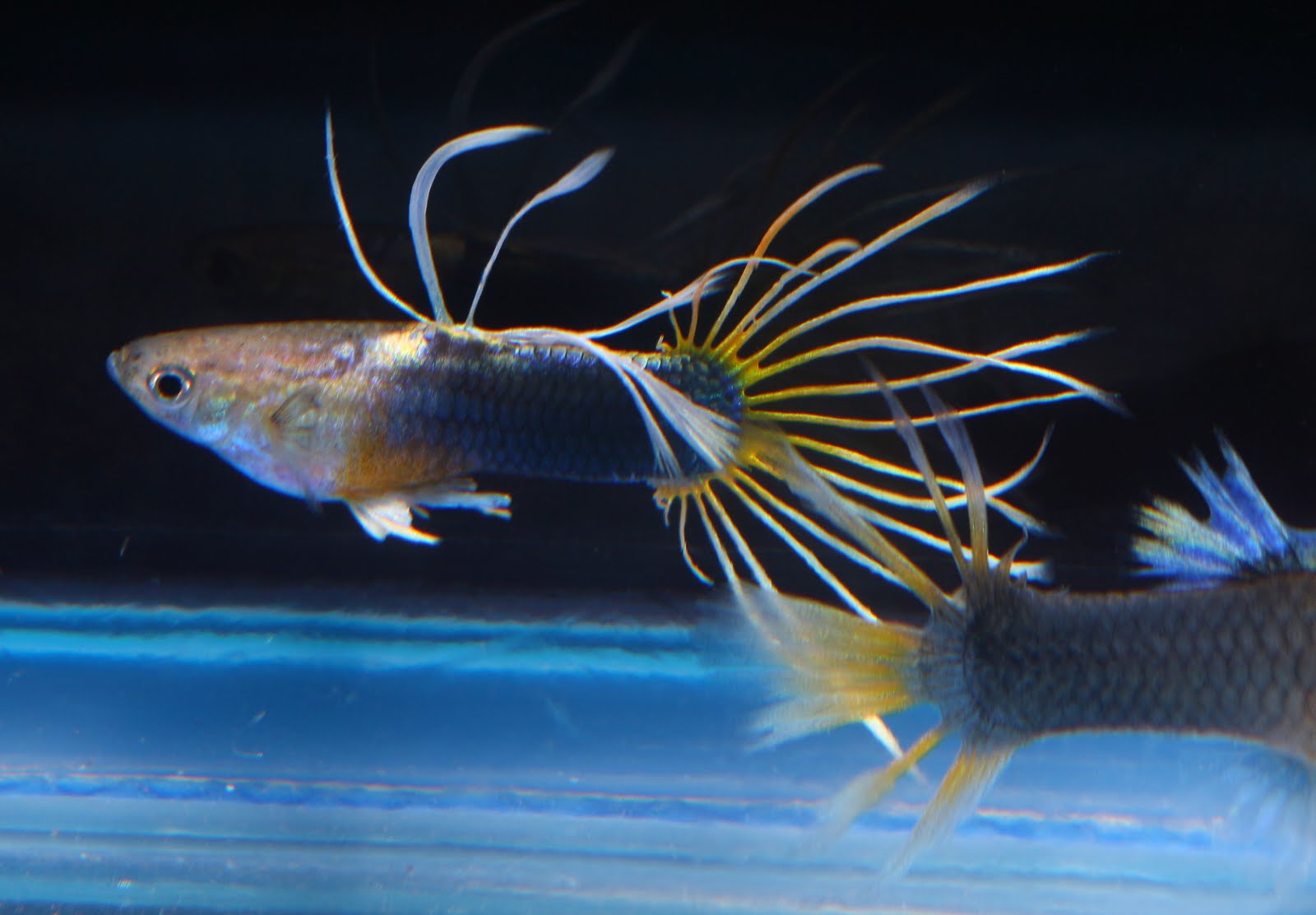An underwater photograph features two distinctive fish swimming against a stark, dark background that transitions to a lighter blue hue at the bottom. The central fish, slightly left of center, displays a light gray head with a prominent black eye and swims to the left. Its body transitions from light to darker gray with an orange tint on its underbelly. Notable are its various fins and unique, long white filaments: some arch upward and curve right, with additional filaments extending in various directions from its midsection and tail. The tail itself showcases an elaborate array of yellow-based, light-colored filaments, some tipped with orange.

On the bottom right, partially extending out of the frame, is the back half of another fish. This fish exhibits a gray body accented with blue, feathery dorsal fins, and a fan-shaped tail marked by yellow at the base and white at the tips. The consistency and lighting of the image suggest it is taken underwater, capturing the intricate and colorful details of these two marine creatures amidst a dark, almost nocturnal aquatic environment.